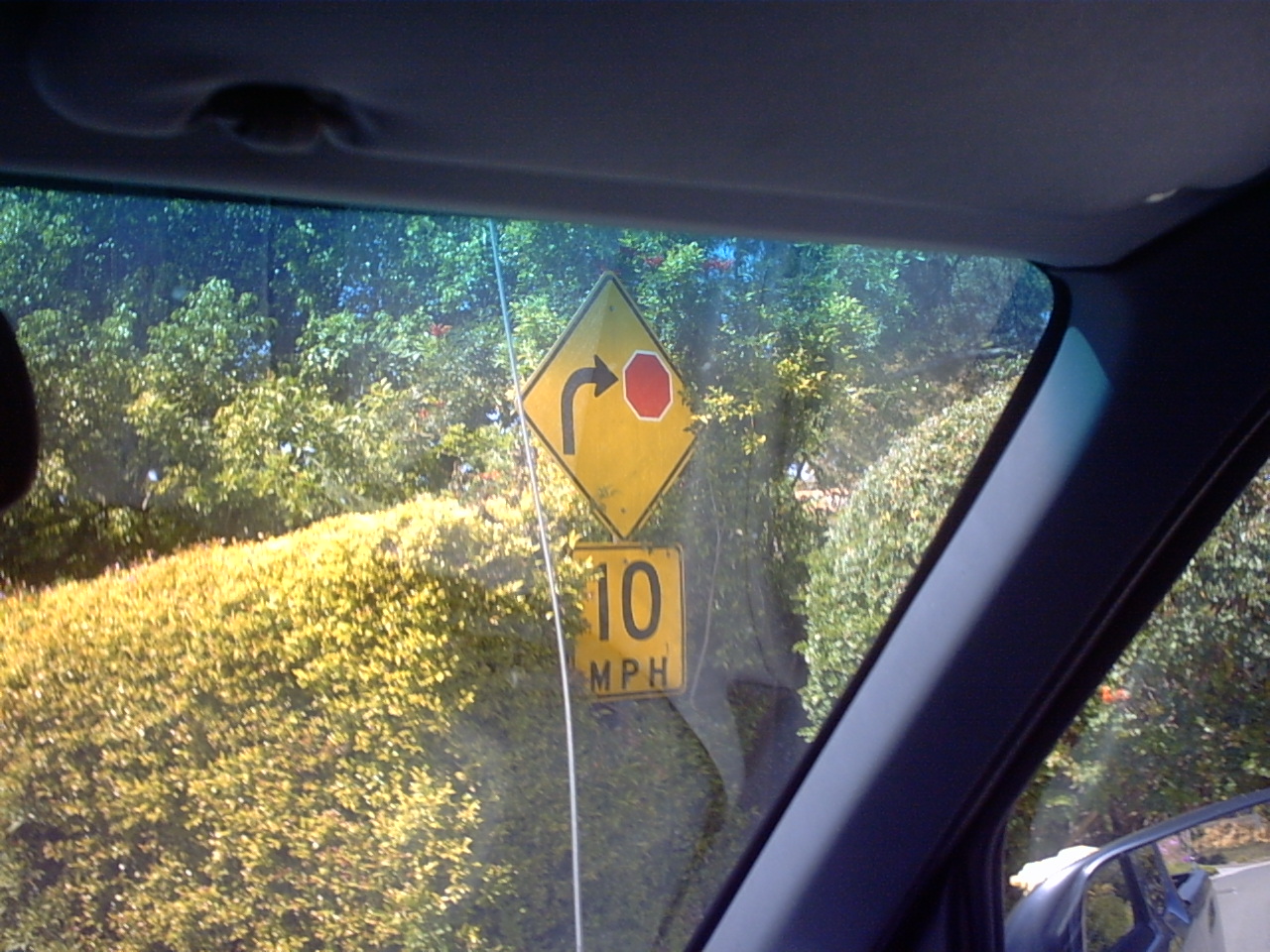This photograph, taken from the upper right corner of a vehicle's front windshield, captures an outdoor scene marked by lush greenery and notable road signage. The backdrop consists of tall green trees, with variations in leaf shades, and a manicured hedge to the left. Framed by the car's dark gray interior, gray roof and visor, and the blue-tinted top edge of the windshield, the focus is a prominent yellow warning sign centered in the image. This diamond-shaped sign, bordered in black, features an upward arrow curving sharply to the right toward a stop sign symbolized by a red hexagon with a white outline. Directly below, a smaller, almost square yellow sign bordered in black indicates a speed limit of "10 MPH", warning drivers to slow down for the approaching curve and stop sign. The lower right of the photo shows the top and left edge of the passenger side mirror, hinting at the vehicle's dark gray interior, possibly that of a small pickup truck. The well-maintained hedge and towering trees behind the sign suggest a residential area.